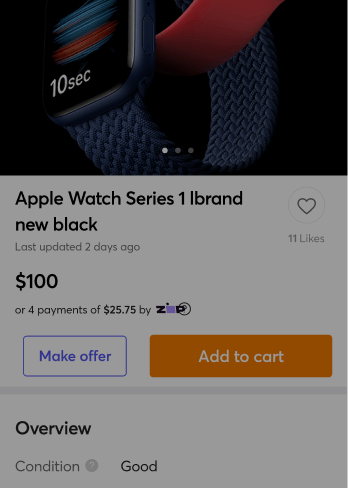A detailed image caption for the Apple Watch Series 1 in New Black:

The image features an Apple Watch Series 1 in New Black, prominently displayed at the top. The watch is equipped with a wristband that appears to be woven, though it may be made of a plastic material. The watch face currently displays a timer set to 10 seconds, indicating the device's functionality.

Below the main image, there are three dots signifying additional images can be viewed by sliding, allowing a more comprehensive view of the product. The listing indicates that the item was last updated two days ago and has garnered 11 likes. There is a heart icon beside the likes count.

The price is marked at $100, with an option to make four payments of $25.75 through Zimp. Users have the option to make an offer via a link in blueish-purple print. For those ready to purchase, there is an orange "Add to Cart" button prominently displayed.

Below these options, a slim gray rectangle separates the purchase information from the product details. The section titled "Overview" appears in bold black print, followed by the word "Condition" in a slightly less bold font, indicating the watch is in "Good" condition.